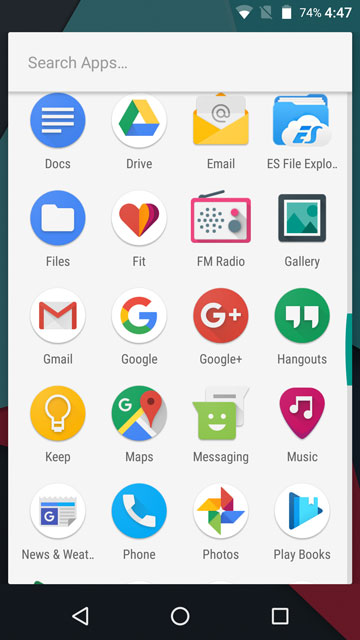Caption: 

A detailed screenshot of a smartphone screen displaying the "All Apps" page in alphabetical order. The status bar at the top right corner indicates the time as 4:47 PM and the battery level at 74%, accompanied by the battery icon. Just below the status bar, a "search apps" bar is visible, allowing users to quickly find specific applications. A dark green scroll bar is located on the right middle side of the screen, suggesting that the user is midway through scrolling. The visible apps in this section include Google Docs, Google Drive, a generic email app, File Explorer, Gallery, Hangouts, Music, Playbooks, Photos, Phone, Messaging, Maps, Keep, Gmail, Google Fit, Files, Google+, News and Weather, and FM Radio.